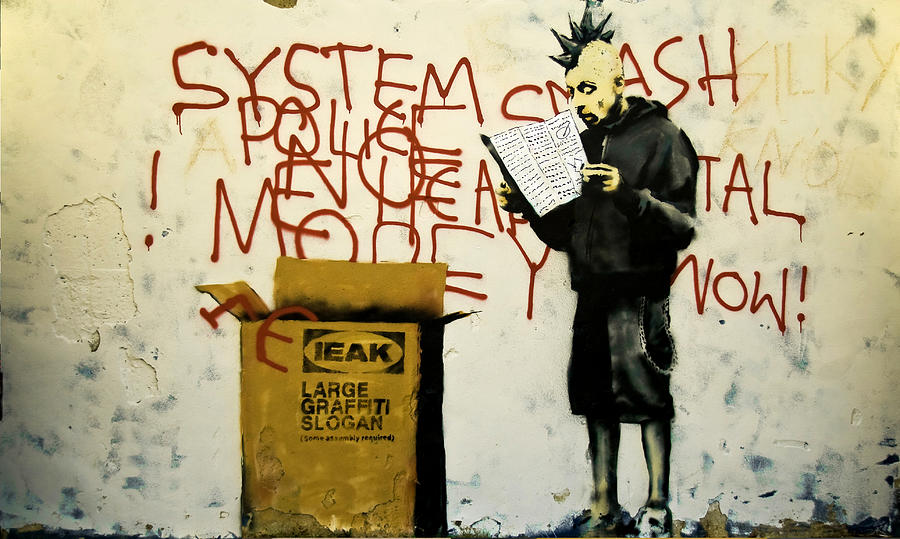The image showcases a vivid piece of graffiti art on the side of a building. Central to the scene is a tall man with a bald head and a spiked black mohawk, wearing a black hoodie, black baggy shorts with a chain, and high-top sneakers. He is intently reading a trifold publication with very small words, his wide eyes suggesting deep concentration. The wall behind him is covered in bold red graffiti that reads "SYSTEM," "SMASH," "POLICE," "NO MORE," "WOW," and other harder-to-read words. Among the chaotic messages, there is an area where letters seem to be tumbling out of a box marked with a logo resembling IKEA’s, but instead labeled "IEAK," with the text below it stating "LARGE GRAFFITI SLOGAN SOME ASSEMBLY REQUIRED." This eclectic mix of elements and rebellious messages captures the raw, punk aesthetic of the street art scene.